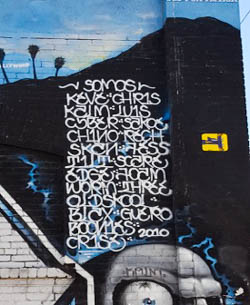The image depicts a mural painted on a brick wall, serving as both graffiti art and a larger piece of street art. Dominating the background is a dark, nearly black, hill with three distinct palm trees sprouting from it. The upper seventh of the mural showcases a slice of blue sky, providing a stark contrast against the dark hill. The lower left corner includes part of a gray brick house, while the center bottom features a curved, gray structure resembling a dome or perhaps a stylized helmet with a prominently large eye, sparking curiosity about its interpretation. Intricate white graffiti scrawls across the dark hill include phrases in Spanish like "somos," listing names such as Kevin Criss, Justin Chino Roche, and others, possibly the artists behind the mural. A small yellow rectangle interrupts the blackness of the hill on the right side, adding another layer of mystery. The mural includes elements that are hard to discern but collectively contribute to its rich, community-art atmosphere.